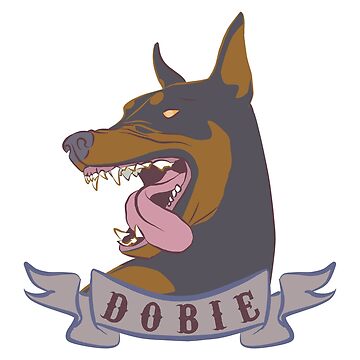The image is a detailed, hand-drawn, cartoonish graphic of a Doberman Pinscher's head and upper neck against a white background, making it appear to float in a white void. The Doberman, primarily black with brown spots around its mouth, neck, and inner ears, has its neck turned, facing left. Its yellow eyes, devoid of pupils, give it a striking appearance, and its open mouth reveals large white fangs, pink gums, and a partially hanging pink tongue, conveying a ferocious snarl. Below the Doberman's neck, a gray banner with a blue border bears the name "Dobby" in brown text, adding a personalized touch to the illustration.